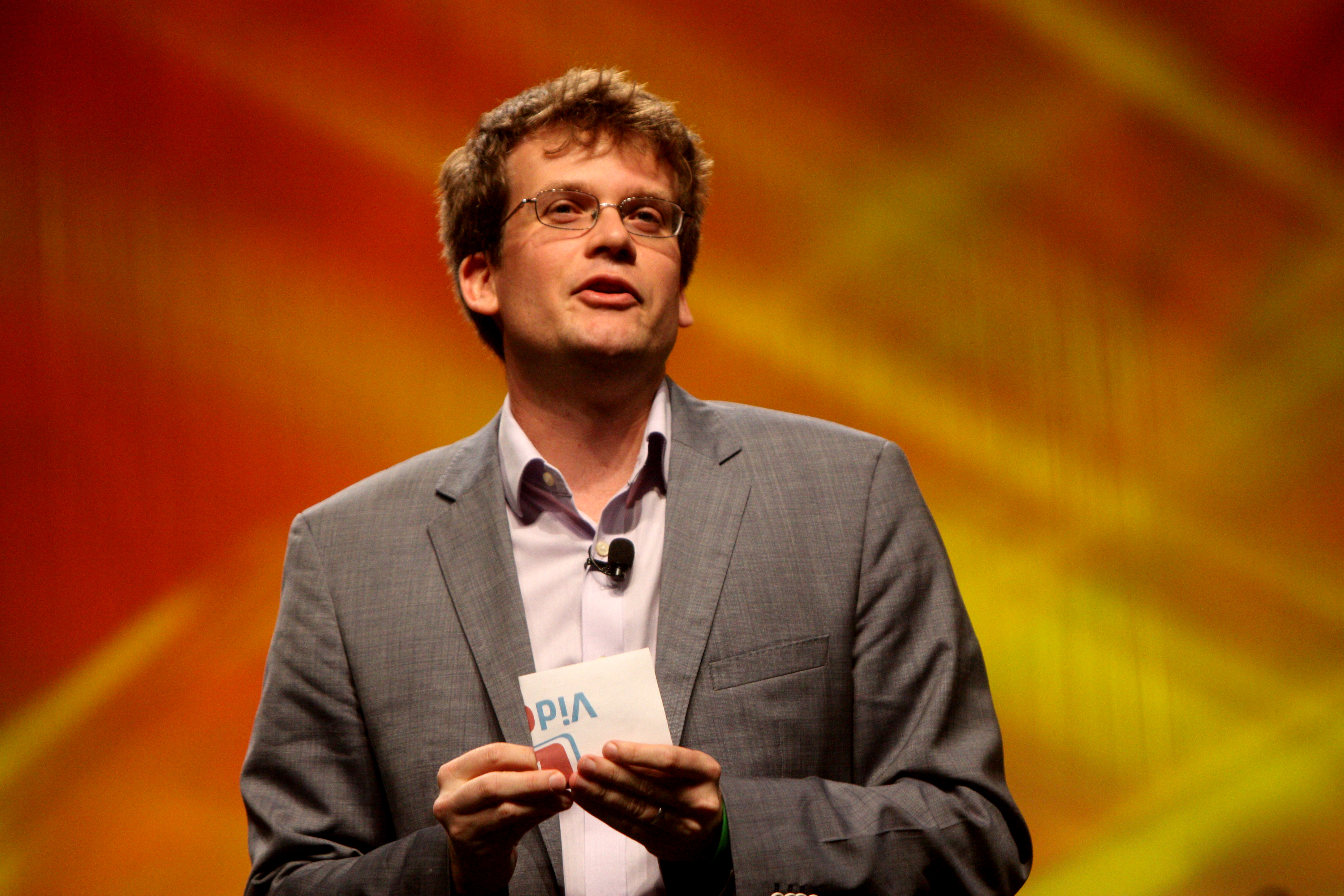This color photograph captures a white man standing on stage, wearing a gray suit jacket over a light tan, possibly light pink or brown, button-down shirt with no tie. He appears to be addressing an audience, indicated by his position and the presence of a small black microphone clipped to the front of his shirt. The background features a vibrant blend of orange and red hues, contributing to the dynamic setting. The man, who sports short brown hair and glasses, is clean-shaven. His hands are close together, holding a piece of paper that displays upside-down letters spelling "V.I.D."